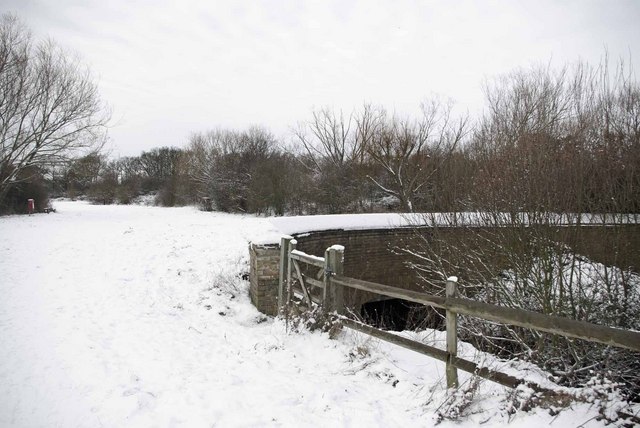The image portrays a serene winter scene with a snowy outdoor landscape. In the foreground, a brick wall runs horizontally, hinting at a possible creek or waterway below. Adjoining the wall on the left is a simple wooden fence, composed of a support post with two vertical beams. A spindly, leafless tree stands beside the fence, echoing the desolation of the winter season. Spanning the bottom half of the picture is a snow-covered field, thinly blanketed and merging into a broader open area. The thick, leafless trees in the background form a dense, skeletal stand under a cold, gray, cloud-filled sky. The predominant colors in the scene are muted whites, grays, browns, and blacks, emphasizing the starkness and stillness of the midwinter setting. The overall ambience suggests a frigid, quiet environment, possibly typical of a rural or forested region like upstate New York.